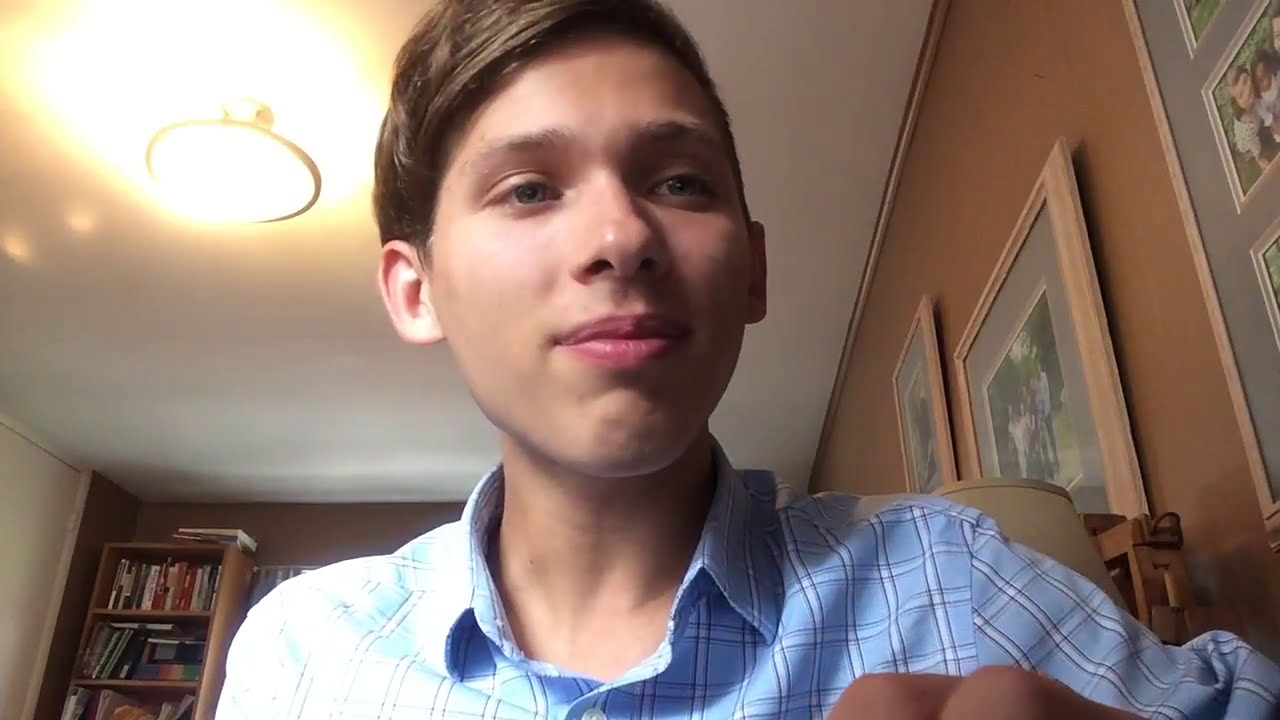The image captures a young boy, around 15 to his early 20s, standing indoors in what appears to be a family room or library. The photo is taken from a bottom-up perspective, revealing a white ceiling with lights on. The room features brown walls with several family pictures hanging and a well-stocked bookcase to the left of the boy. He is centrally positioned in the image, dressed in a blue dress shirt with white stripes, and has blue eyes with brown hair. He appears to be amused, looking off to the right side of the frame. Various colors such as yellow, white, tan, brown, pink, light blue, red, and green are visible, contributing to the warm, vibrant atmosphere of the setting.